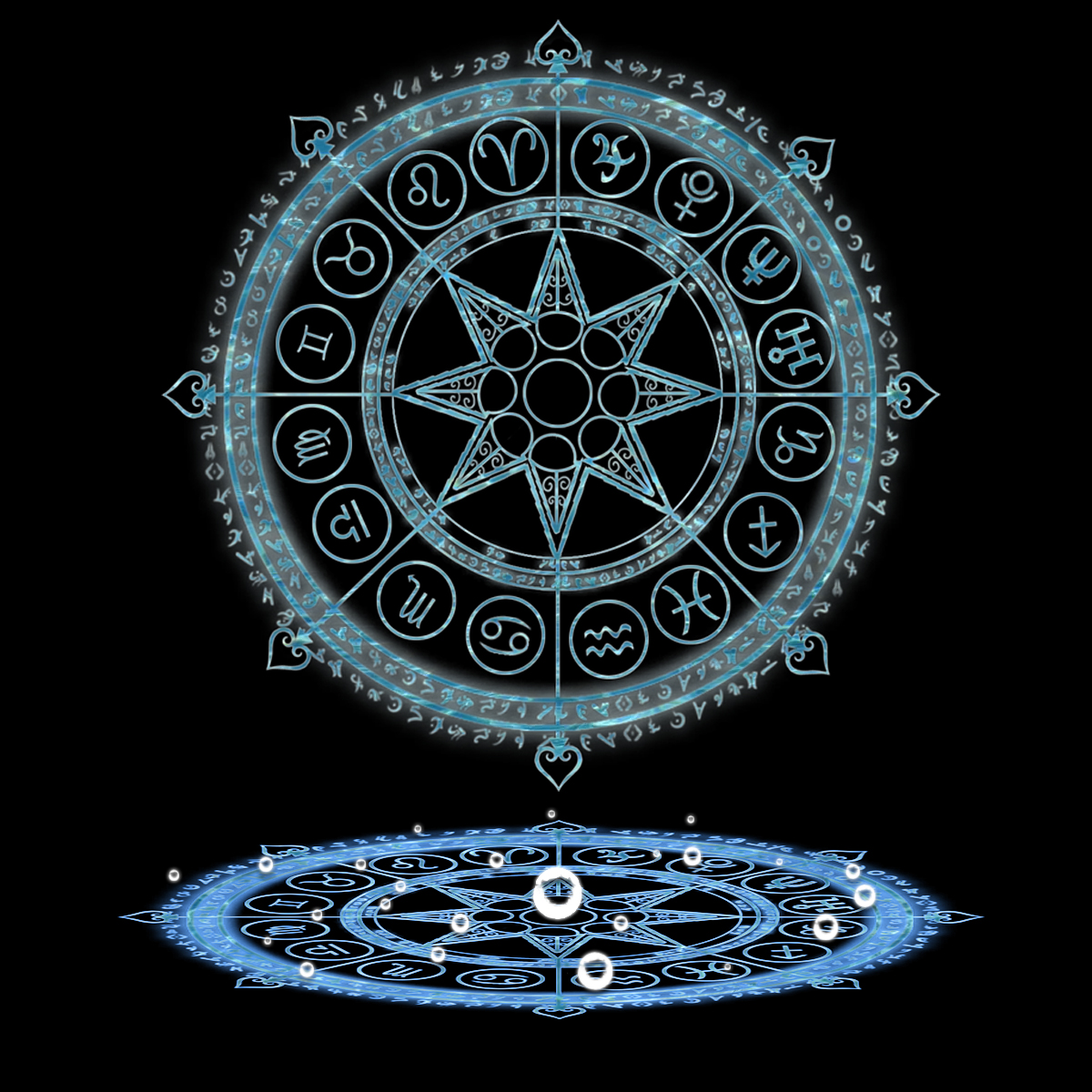The image showcases a large, square composition with a solid black background. Dominating the upper central portion is a large circular design. This primary circle features a border shaded in gray with a light blue outline. Encircling the larger circle are small blue circles, each containing various symbols. At the heart of this design is an eight-pointed star in light blue, with black three-quarter circles around its edges and a central black circle. Extending from each point of the star are lines that end in spade-like shapes at the outer edges. Surrounding this inner structure is a circular band emitting blue light, followed by a broader black band adorned with symbols and round white circles. Another thin, light blue band outlines the entire circle, with additional gray symbols scattered around the circumference.

Perpendicular and lying below this primary circle is a secondary circular design, mirroring the upper one's intricate pattern but in a brighter blue hue. This second circle appears as a reflection or replicated version of the primary design, contributing to a cohesive and symmetrical aesthetic. The overall effect is a detailed and richly symbolic visual arrangement set against a stark black background.